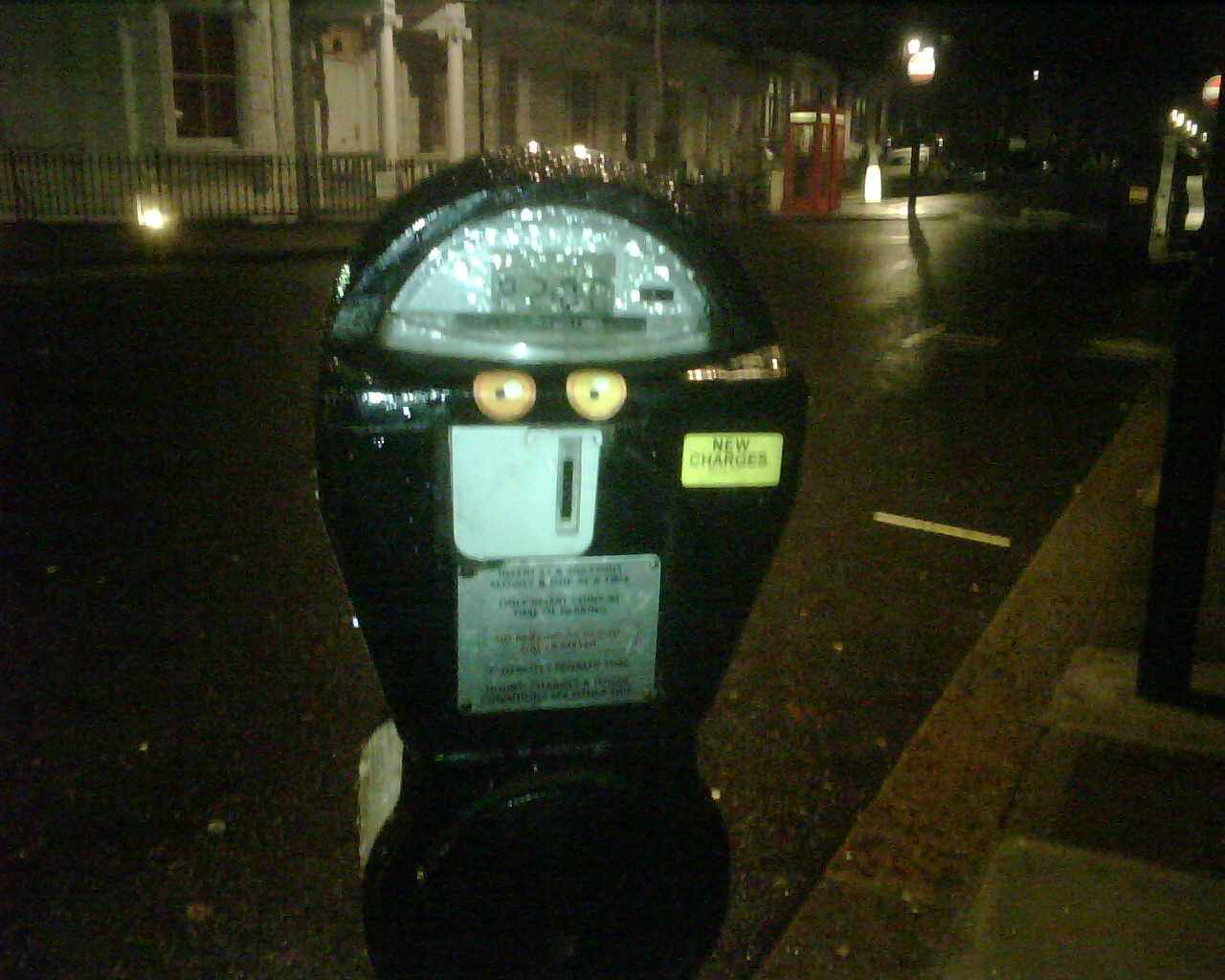The image portrays a nighttime street scene centered on a black parking meter, glistening with rain droplets that obscure the details slightly. The top of the meter features a digital display encased in glass, rendered unreadable by the wetness. Below the display are two yellow circles and a prominent yellow sticker proclaiming "NEW CHARGES" in bold black letters. The meter has a coin slot and a text box with instructions or information that remains indiscernible due to the blur. The background reveals a wet black street, delineated yellow parking lines, a stretch of concrete sidewalk, and a classic red telephone booth reminiscent of old-fashioned London. There's also a hint of a house and street lamps visible through the rainy haze, emphasizing the scene's nocturnal ambiance.